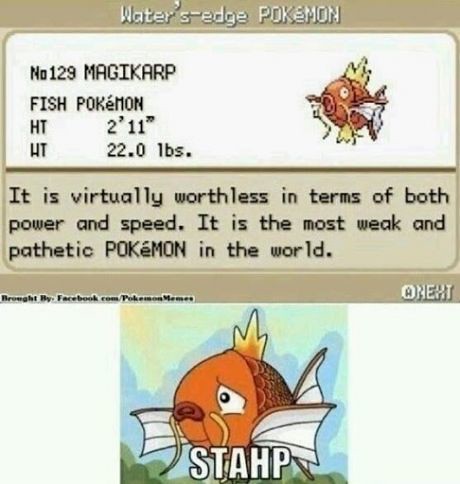The image is a humorous Pokedex entry for Magikarp, the Fish Pokémon, divided into two sections. The top section features a light beige background with the title "Water's Edge Pokémon" in white letters. Below this, on a white background, it lists detailed information in black text: number 129, Magikarp, Fish Pokémon, height 2 feet 11 inches, weight 22 pounds. To the right, there's a pixelated image of an orange Magikarp with yellow and white fins. The entry humorously describes Magikarp as “virtually worthless in terms of both power and speed” and calls it “the most weak and pathetic Pokémon in the world.” At the bottom of this section, there are credits to "Facebook.com Pokémon memes," and an icon indicating to press the A button for next.

The lower section of the image centers on a meme featuring the same orange Magikarp, now frowning. Beneath this image, in white text, it says "S-T-A-H-P." This meme adds a comedic twist to the already humorous Pokedex entry.